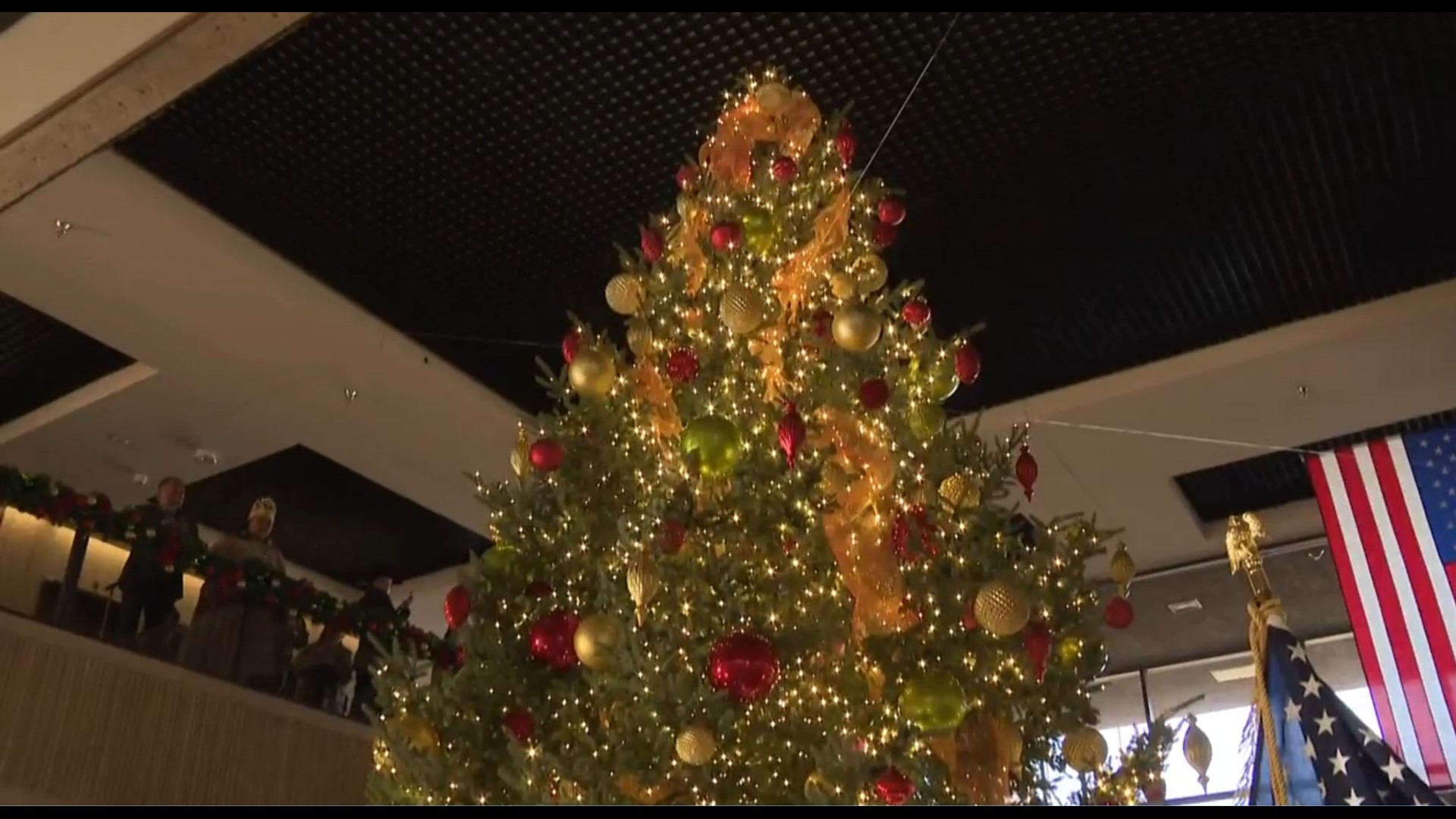This color photograph captures the grand interior of a two-story government building, adorned for the Christmas season. Dominating the foreground is a towering Christmas tree, lavishly decorated with red, green, and gold ornaments, sparkling with lights and gold garland. The tree’s impressive height reaches up to the second floor, where it is anchored by strings for stability. To the left of the tree, a railing draped in festive decorations is visible, behind which stand a couple of onlookers. On the right side of the image, two American flags are prominently displayed—one hanging vertically from the ceiling and the other mounted on a flagpole topped with a golden eagle statuette. The photograph captures the season’s festive atmosphere within a classic government setting, merging traditional holiday cheer with a sense of national pride.